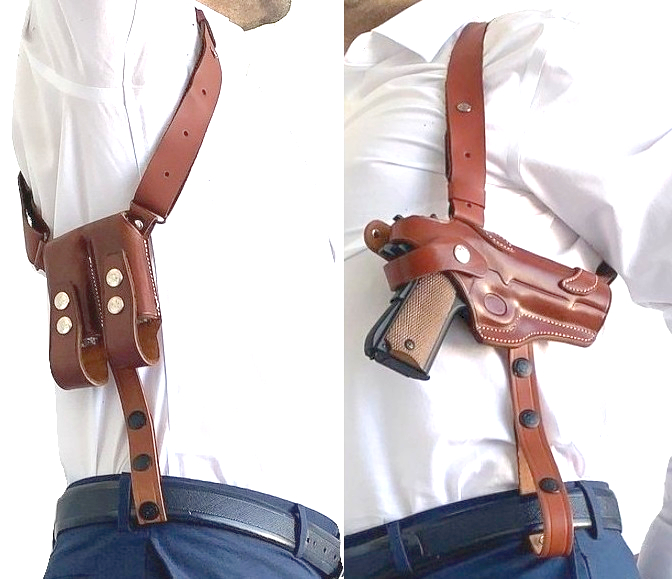The image is a detailed photograph showcasing a man dressed in dark blue pants, a white shirt with a collar, and a black belt, wearing a brown leather underarm gun holster. There are two side-by-side pictures: the left side features an empty holster segment that is connected loosely with straps going around the man's shoulder and fastening to his belt that helps secure it. This side has compartments for holding gun magazines, tightened with buttons and pins. The right side of the image displays another close-up of the holster under the man's left arm, which includes a black and brown gun inserted horizontally into the brown leather harness.